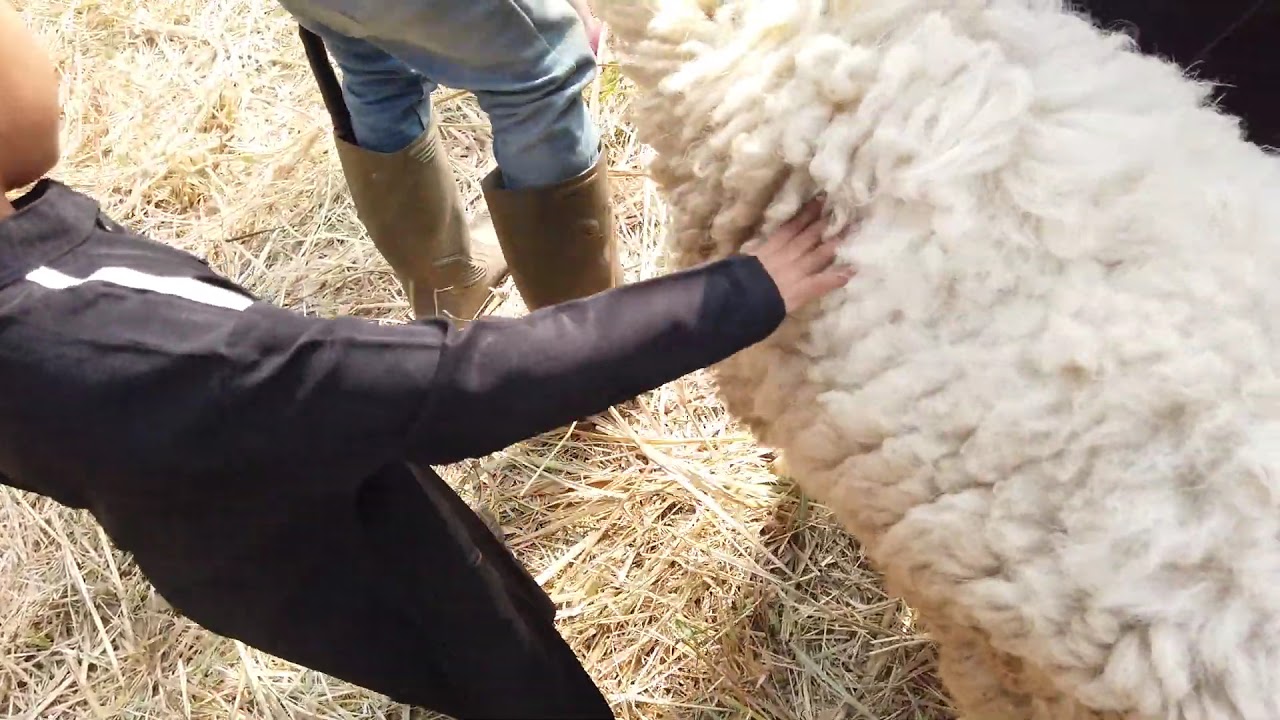In this image, a small child is petting a fluffy white sheep, predominantly showing the sheep's wooly back without its head visible. The child, whose face is partially seen, is wearing a black long-sleeved shirt or jacket with dark pants. His right hand is immersed in the sheep's deep, matted fur, indicating a tactile moment of interaction. He stands amidst a ground covered in golden straw, illuminated by natural sunlight, suggesting an outdoor setting. Directly in front of the child, a person, possibly an employee of the petting zoo, stands wearing light blue jeans and greenish-tan rubber boots. Notably, there is an object, such as shears or a machete, tucked into this person's left boot, hinting at farm-related activities. The overall scene exudes a rustic, farm-like atmosphere, typified by its sunlit, straw-covered ground, with a black object faintly visible in the top right corner of the image.